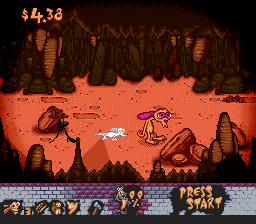The image resembles a scene from a video game or a cartoon panel. At the top left corner in orange text, the number "$4.38" is displayed. Dominating the bottom of the image is a gray brick wall, with bricks partially descending in the center, revealing a black background. Within this section are various icons, including what appears to be a cat's head in black cutout forms, yellow numbers "3" and "99%", and possibly another cat head in orange. To the right, in an orange font, the words "Press Start" are prominently featured. In the central part of the scene, a small orange cat with distinct pink eyes and ears is fleeing from a small white mouse along a dirt path. Flanking the path are dark rock formations, suggesting a cave-like environment. A dazed beige rabbit with long drooping purple ears and large purple eyes stands off to the side, its palms facing upwards, gazing blankly into the distance as if in a trance. The ground appears clay-like, reminiscent of the surface of Mars.